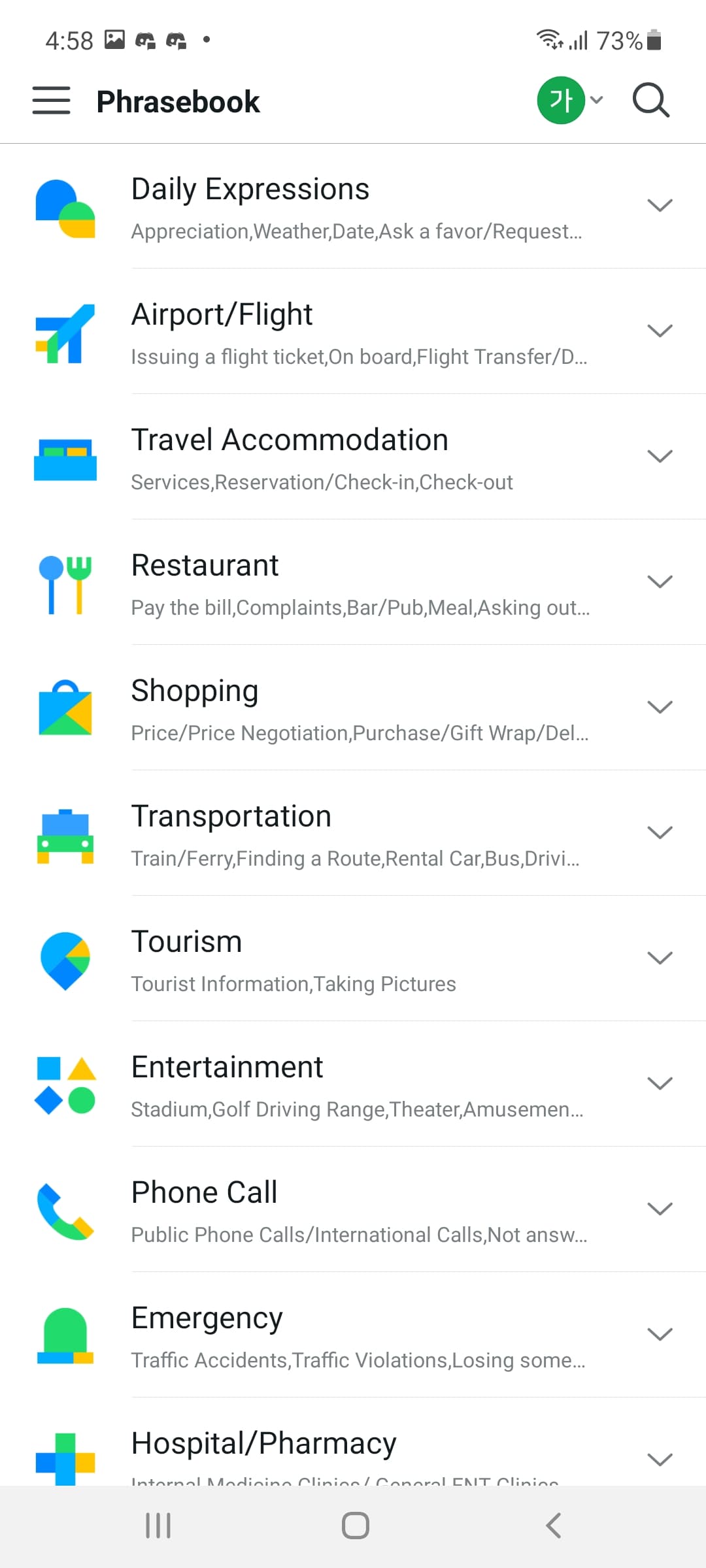A screenshot from a very tall and narrow mobile phone display, approximately 3.5 to 4 times taller than it is wide, captures an interface from an app titled "phrasebook." The presence of mobile reception bars, a 73% battery life indicator, a Wi-Fi signal icon, and the time displayed as 4:58 (ambiguous whether a.m. or p.m.) confirms that it's taken from a phone.

The top-left corner features the app's title, "phrasebook," written without any spacing. On the upper-right, a green circle contains an Asian character, indicating that the phrasebook likely caters to this particular language. 

The main content area is organized into different categories, each with an icon taking up about 15% of the screen width on the left. The top category is named "Daily Expressions," featuring subcategories like appreciation, weather, date, and ask a favor/request. To the far right of the "Daily Expressions" category is a down arrow, suggesting that clicking it would reveal more phrases.

Following "Daily Expressions," other categories listed include "Airport/Flight" with helper text such as "issuing a flight ticket, on board, flight transfers," accompanied by an airplane icon. Additional categories cover various aspects of travel and daily life, including "Travel Accommodations," "Restaurants," "Shopping," and "Transportation." The consistent primary color scheme of blue, green, yellow, and shades of blue is used throughout the icons for these categories.